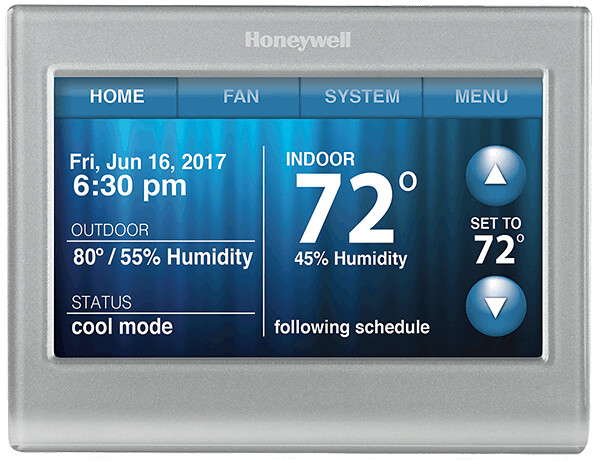This image is a professionally captured photo of a Honeywell digital thermostat, likely sourced from an e-commerce website. The device features a sleek, silver rectangular design with the brand name "Honeywell" engraved at the top. The large, digital screen displays multiple sections, indicating its sophisticated, all-digital functioning system. At the top of the screen, there are four selectable categories: "Home," "Fan," "System," and "Menu."

The screen shows detailed information including the date and time—Friday, June 16th, 2017, at 6:30 p.m. Additionally, the outdoor temperature is displayed as 80 degrees Fahrenheit with 55% humidity. The current operation mode is set to "Cool." On the right-hand side of the display, the indoor conditions are provided: 72 degrees Fahrenheit with 45% humidity. Below this, two circular buttons with up and down arrows allow for manual temperature adjustments. Positioned between these buttons, the current set temperature is indicated as 72 degrees, and the mode status is listed as "Following Schedule" in white text.